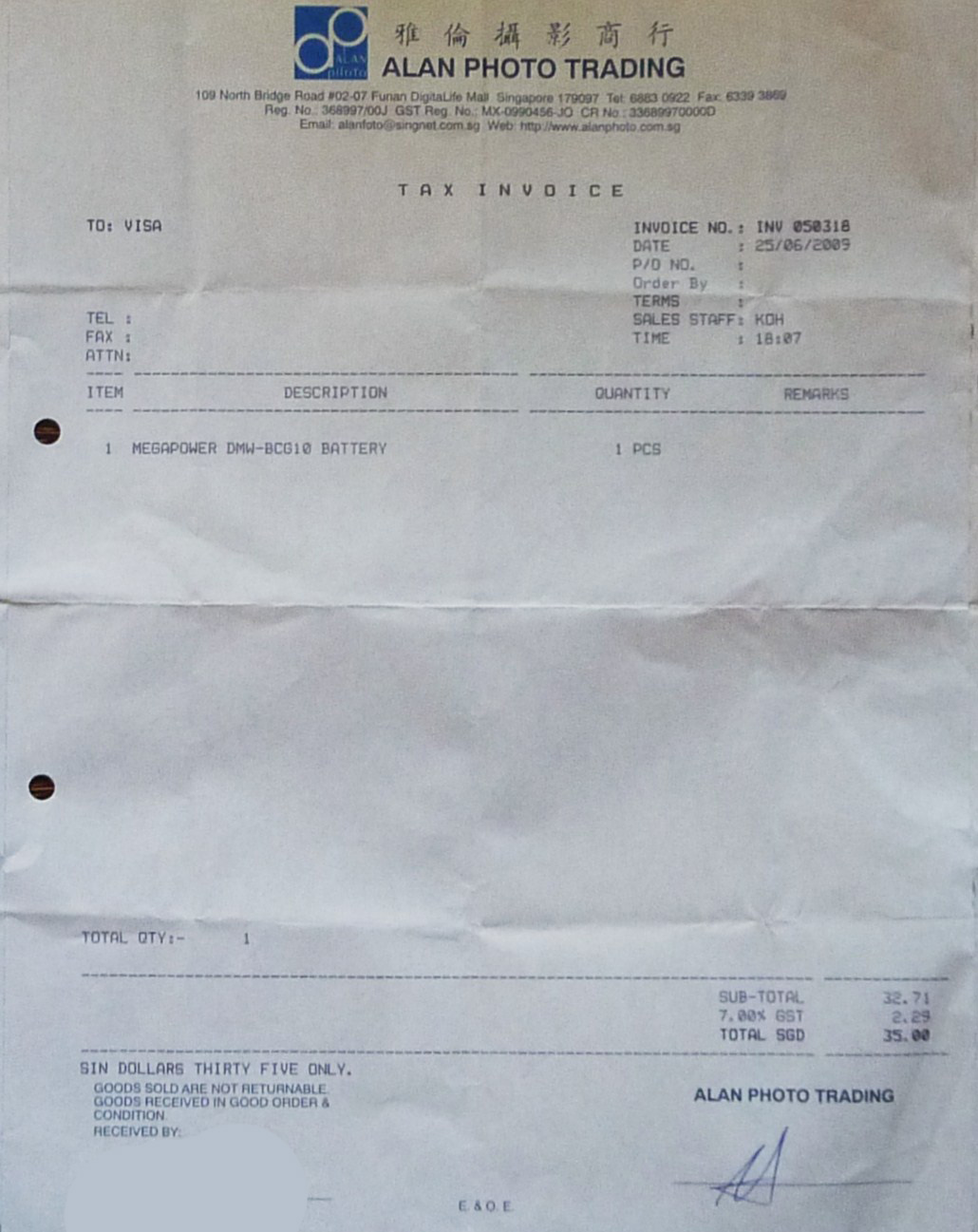This image displays a detailed receipt printed on white paper with black ink. At the top of the receipt, "Allen Photo Trading" is prominently featured, accompanied by a blue and white logo. The document is marked as a tax invoice made out to Visa, bearing the invoice number 050318. The transaction date is June 25, 2009. Beneath the basic information, there are additional details, including the total purchase amount of $35. At the bottom of the receipt, both the signature of the individual who signed the receipt and the sales staff ID are clearly visible.